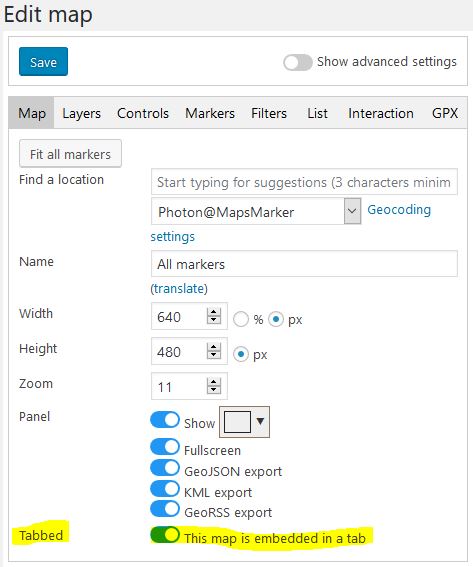In the upper left corner, there is the text "Edit Map." Below this, to the left of the next rectangle, a blue box contains the word "Save." To the right of this, the text "Show Advanced Settings" appears with a circle to the left in the gray bar. Just below, "Map" is highlighted in a gray square, and to its right, there are various options listed: "Layers," "Controls," "Markers," "Filters," "List," "Interaction," and "GPX."

Beneath this section, another rectangle contains the phrase "Fit All Markers." Below this, in black text, is "Find a Location," accompanied by a search bar. Inside the search bar, it prompts "Start typing for suggestions (three characters minimum)." Further down, the text "Photon at Maps Marker" is displayed, with the adjacent blue text "Geocoding Settings."

To the left side, the word "Name" is visible, followed by a rectangle labeled "All Markers Inside," and below this, in parentheses, it states "(Translate)." Extending all the way down to the lower left corner, the word "Tabbed" is highlighted in yellow. Also highlighted in yellow is the phrase "This map is embedded in a tab."